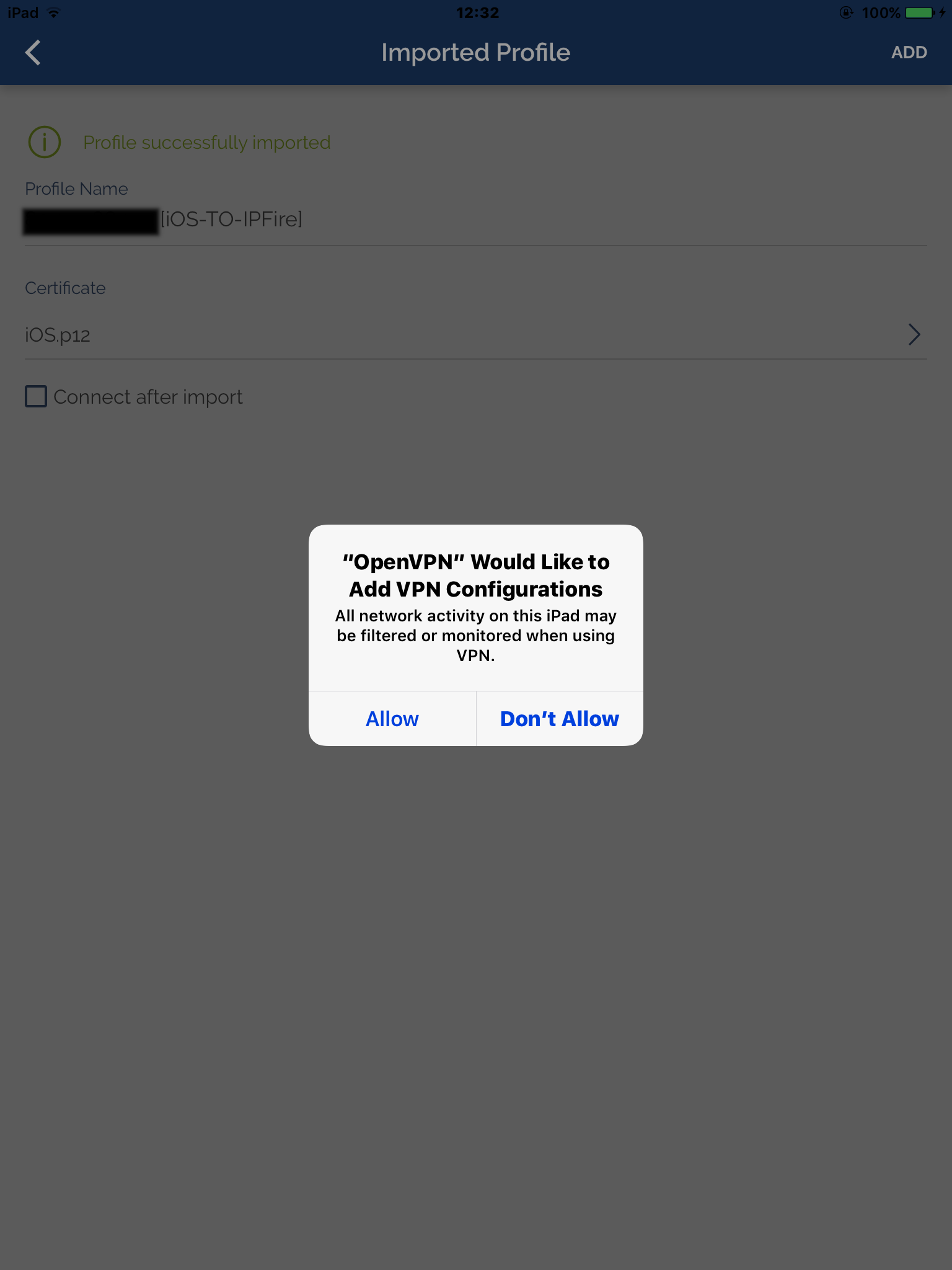A darkened screen displays a pop-up in the middle, resembling a phone or iPad interface with a vertical orientation. The central white pop-up, featuring rounded corners, contains black bold text reading “OpenVPN” in quotation marks, with the message: “would like to add VPN configurations.” Below this, smaller black text states: “All network activity on this iPad may be filtered or monitored when using VPN.” Two buttons are present below the text: “Allow” in blue on the left and “Don’t Allow” in darker, bold blue on the right.

The background reveals contextual details at the top of the screen: on the left, black text displays "12:32," and to the right, a 100% battery icon with a green fill. A blue area beneath this shows white text reading “Imported Profile,” accompanied by a white arrow pointing left and the word “Added” on the right. Below this, a page confirms: “Profile successfully imported” with the profile name obfuscated as "liOS-to-IPFIR." Additional details include a certificate file "liOS.p12" and an unchecked option labeled “Connect after import.”